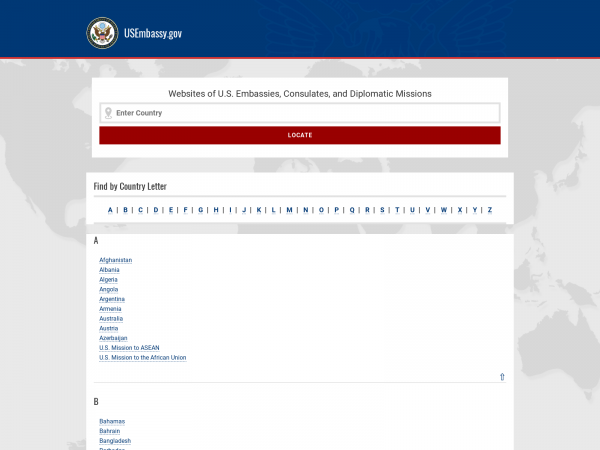The image displays a detailed interface of the USEmbassy.gov website, set against a striking purple background with subtle map features. At the top left, there is a dark purple square housing an emblem of an eagle inside a circle, accompanied by the text "USEmbassy.gov." Below the emblem, the webpage prominently features a large white box with the title "Websites of U.S. Embassies, Consulates, and Diplomatic Missions."

Further down, there's an input field labeled "Enter Country," followed by a red "Locate" button. Adjacent to these, another large white box is labeled "Find by Country Letter," which provides an alphabetical list from A to Z in blue, each letter separated by small lines. A drop-down menu appears under the letter "A," listing countries such as Afghanistan, Albania, Argentina, and Australia. Similarly, the letter "B" follows with a list of B countries. Between the sections for the "A" and "B" countries, a small, indistinguishable blue character is visible.